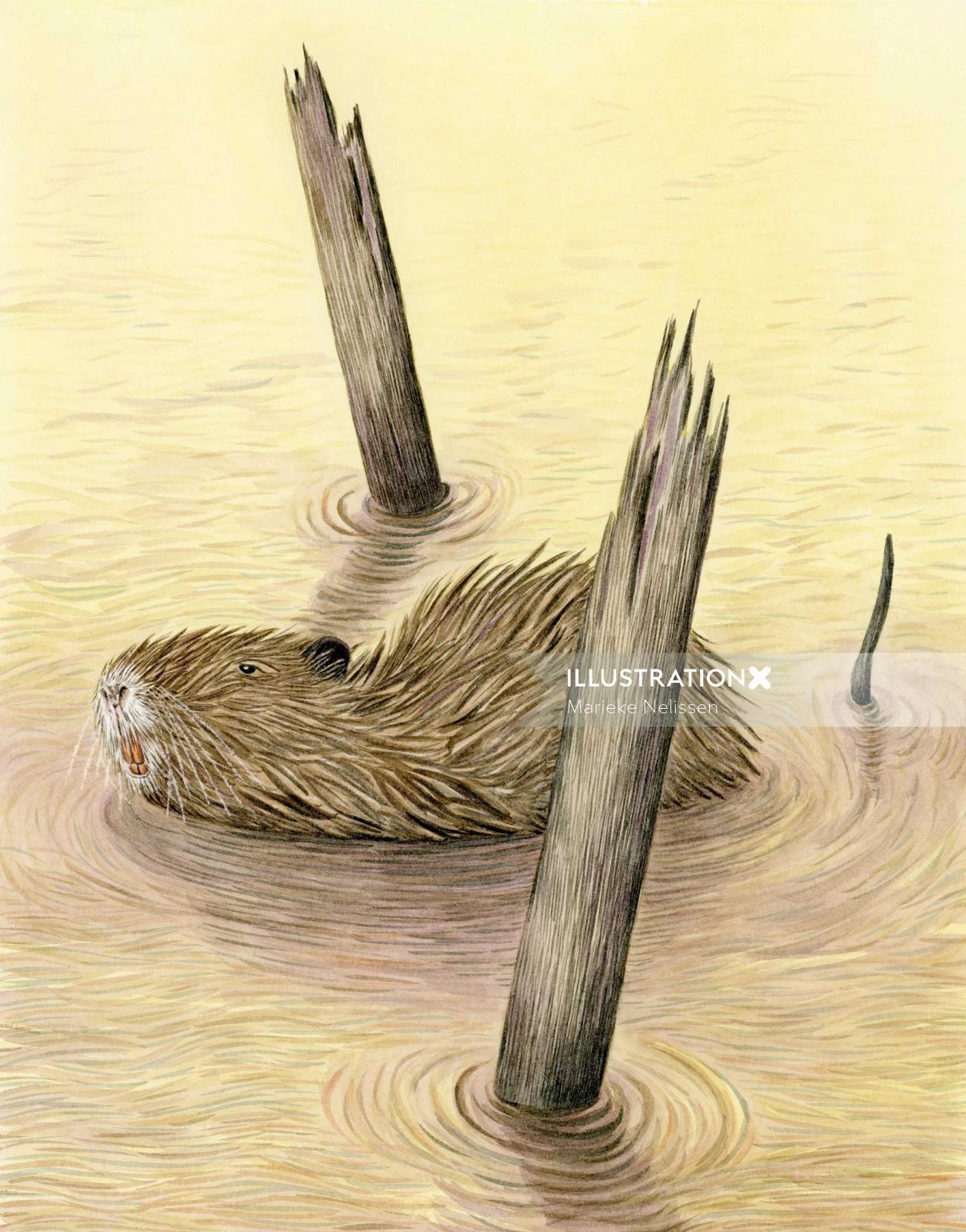The image depicts an illustrated aquatic mammal, likely a beaver or an otter, swimming in yellowish-tan water. The creature features wet, light brown fur, prominent long yellowish teeth, and a notable white region around its nose. Its thin, black tail, resembling a rat's tail, is also visible protruding from the water. Surrounding the mammal are broken tree branches or logs, sticking out of the water, creating ripples across the surface. The illustration is tagged with an ink mark that reads "Illustration X" overlaying the scene.